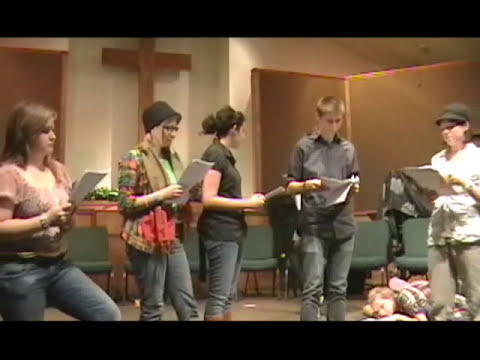In this image, five teenagers—four girls and one boy—are standing in a semi-circle, holding pieces of paper, possibly sheet music or scripts, and looking down at them. They seem to be engaged in a choir practice or a skit rehearsal, set in a church-like environment. Behind them are green chairs arranged in a semi-circle and a white wall adorned with a large wooden cross, adding to the chapel ambiance. The teenagers are equally spaced in the foreground, showcasing a variety of clothing colors: the first girl, with brunette hair, wears a light pink shirt and denim jeans; the second girl, sporting glasses and a black hat, has on a plaid shirt, scarf, and denim jeans; the third girl wears a black short-sleeved shirt with her hair in a messy bun and denim jeans; the boy is in a gray button-down shirt with blonde hair and denim jeans; and the final girl on the right, wearing a black hat, is dressed in a white button-down shirt and khaki pants. The overall scene suggests an informal yet focused practice session, with the cross symbolically overseeing their activities.